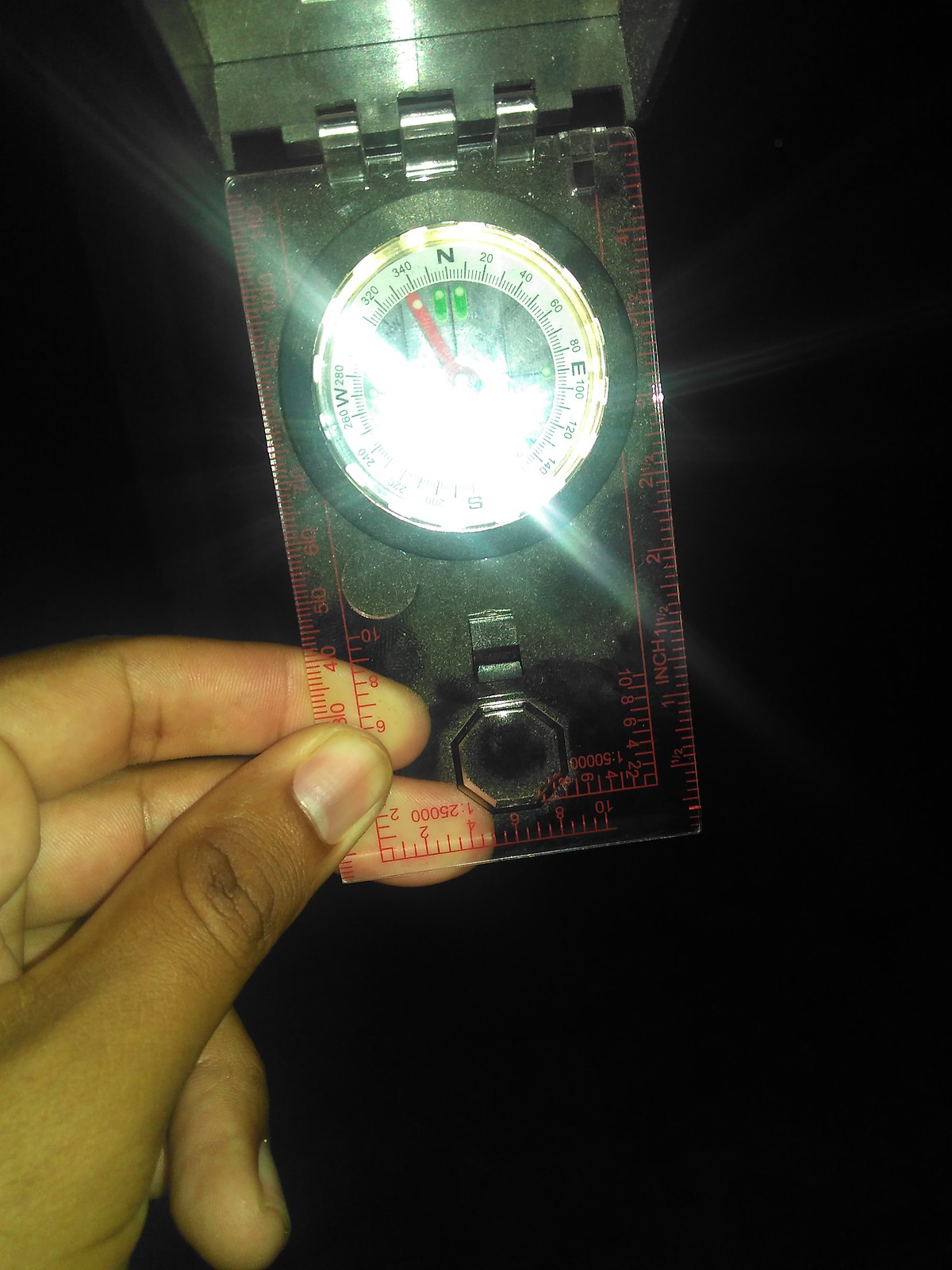A captivating photograph depicts a person with dark skin, possibly of Indian descent, holding a clear acrylic compass. The compass, designed to be laid on a map for navigation, is held steadily by the subject. A bright light shines from behind, illuminating the compass and creating a mesmerizing display as it passes through the glass bubble encasing the needle. The needle, pointing nearly north but off by a degree or two, serves as the central focus. This light refracts through the bubble, casting multiple beams in various, captivating directions, with two prominent beams in stark opposition. Smaller, scattered light patterns add to the enchanting visual effect. The background is completely black, hinting that a flashlight may be used to produce this striking illumination and to emphasize the intricacies of the compass and its refracted light.